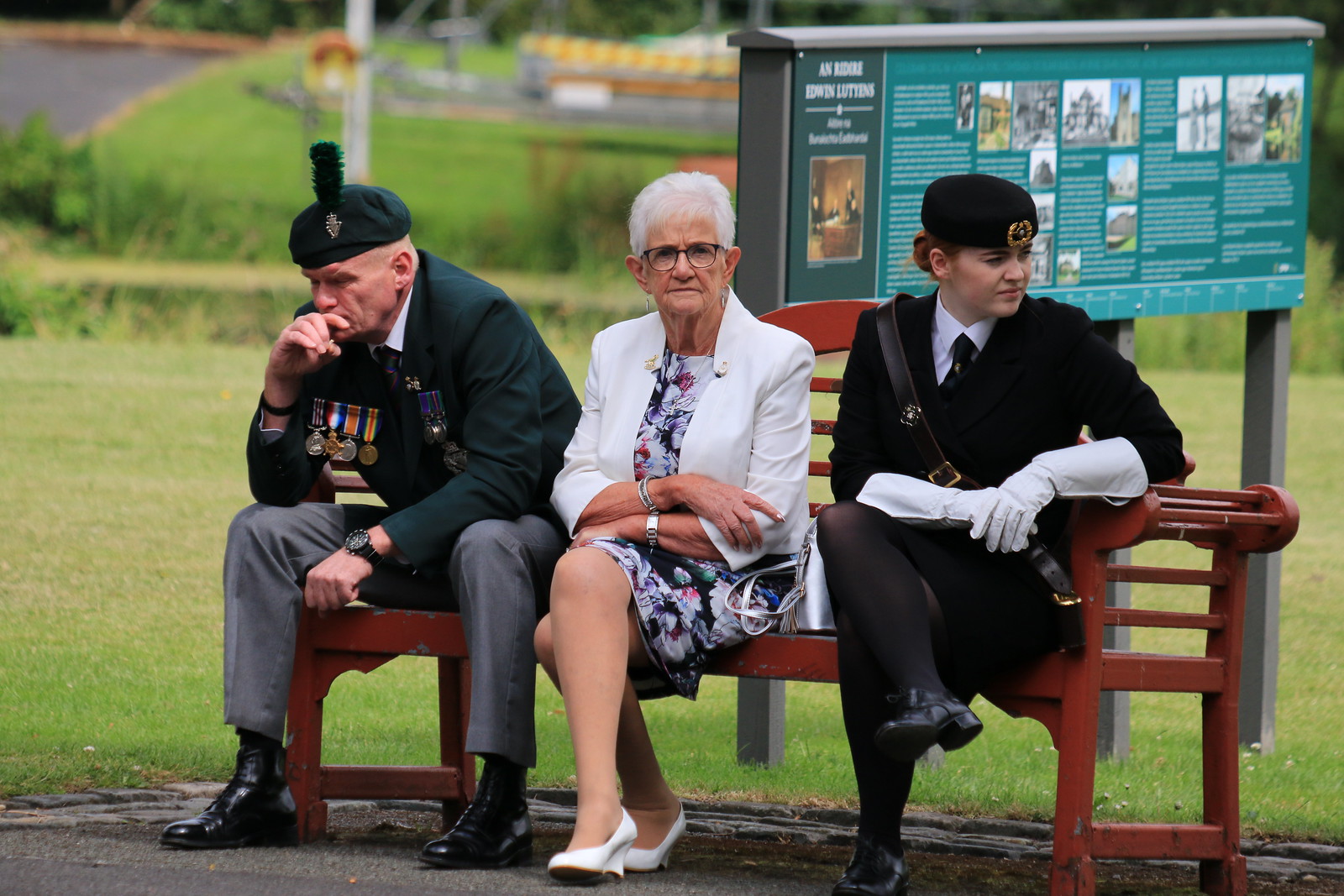In this detailed image, set outdoors, you see three individuals sitting on a wooden brown bench set against a backdrop of an expansive grassy area that fades into the distance and includes a blurred information board with partially readable text. On the left, there's an elderly gentleman dressed in a dark military suit accessorized with a beret that has a black feather at the front. His attire includes a dark military jacket adorned with medals on his right chest, gray pants, and black boots. He is leaning forward with his elbow on his knee, his hand covering his mouth as he gazes intently at the ground. In the center, there is an elderly woman with short white hair and glasses, wearing a white suit jacket over a black and white flower-patterned dress, and white pumps. She has a stern expression and her arms are crossed over her body. To the right, a younger woman dressed in a black suit jacket, white shirt, black tie, black skirt, and black shoes, sits with her legs crossed. She also sports a black beret with a badge and white gloves, and she looks off to the side.